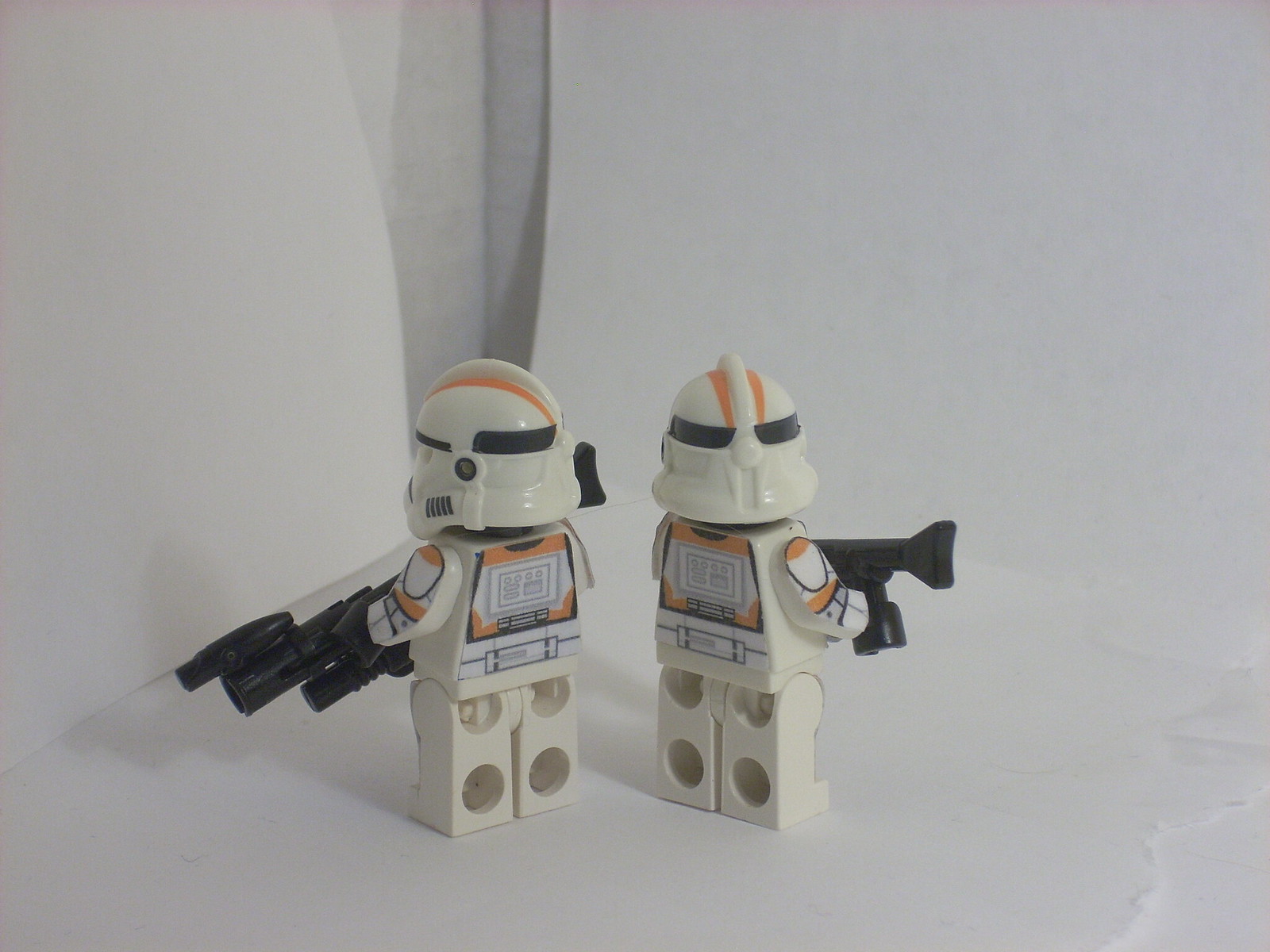This indoor photograph features two Lego Star Wars figurines, specifically stormtroopers, standing side by side with their backs turned to the camera. The figurines are clad in detailed white armor adorned with orange accents, including stripes on their helmets and shield-like designs on their arms. Each stormtrooper holds a substantial black futuristic gun. The scene is meticulously staged against a plain white backdrop, created by torn sheets of paper arranged to resemble snow or a minimalist landscape. The edges of the torn paper are visible in the bottom right corner of the image. The surface they stand on is also white, presumably matching the white table beneath. The helmets of the figurines are distinctive, featuring a crest in the center and horizontal black strips for the visors. The figurines have characteristic holes in the back of their legs, designed to connect with other Lego blocks. There are no other objects or characters present, making the image solely focused on these two figures.